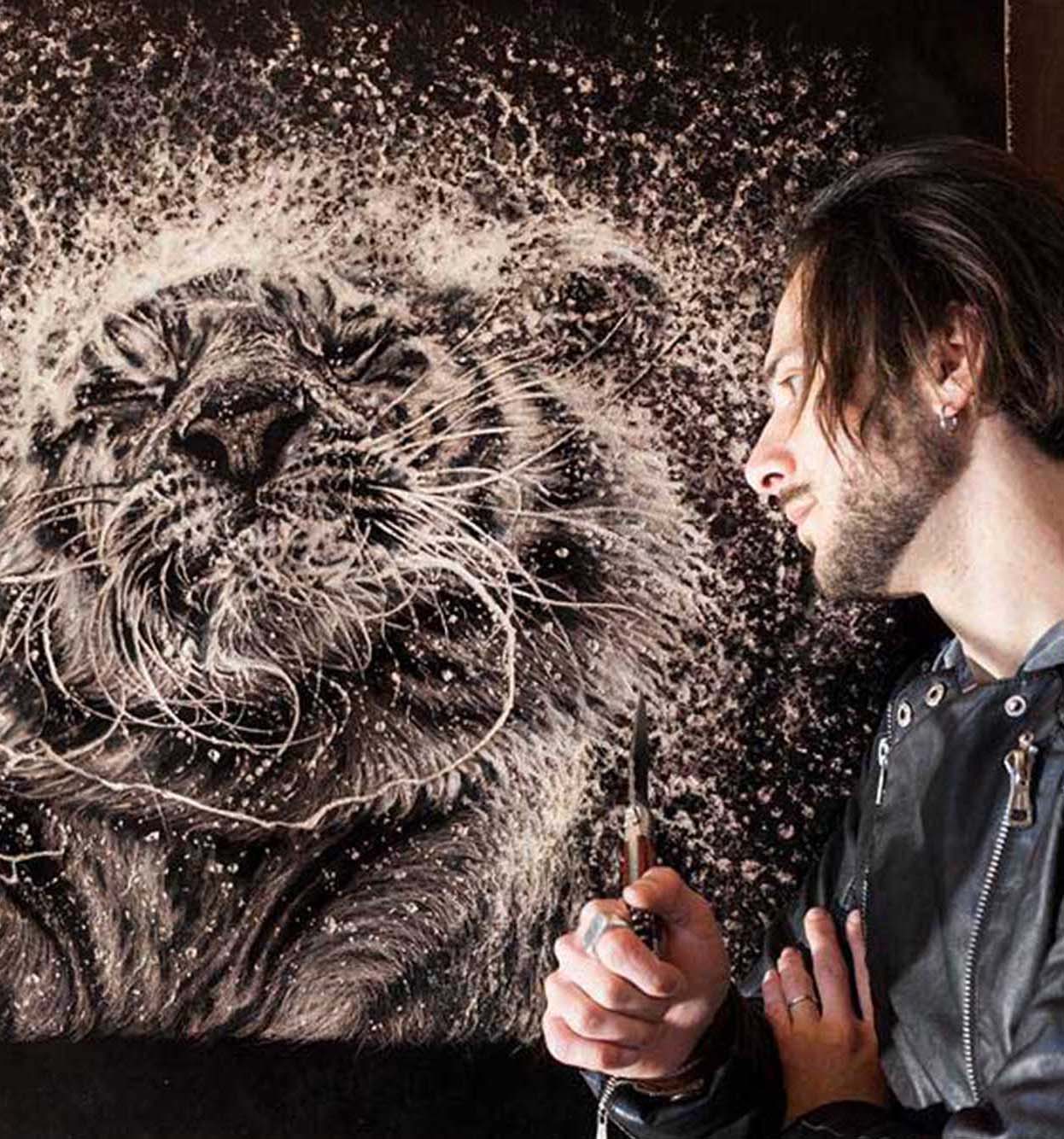This square image depicts a man intently working on a painting. Positioned to the right-hand side, only part of his figure is visible, showcasing his long black hair, thin short beard, and a hoop earring in his left ear. He wears a black leather jacket, with his left hand resting on his right arm, revealing a wedding ring. In his right hand, he holds an object that resembles a pen or possibly a sculpting tool or scalpel. The painting he is focused on features a striking, computer-generated image of a lion or tiger's face, composed of dynamic black and white, and whitish-tan colors. The animal's features, such as its nose and stripes, are distinctly visible, while the rest of the image appears scattered and splattered, creating a starry or explosive effect on the dark background.